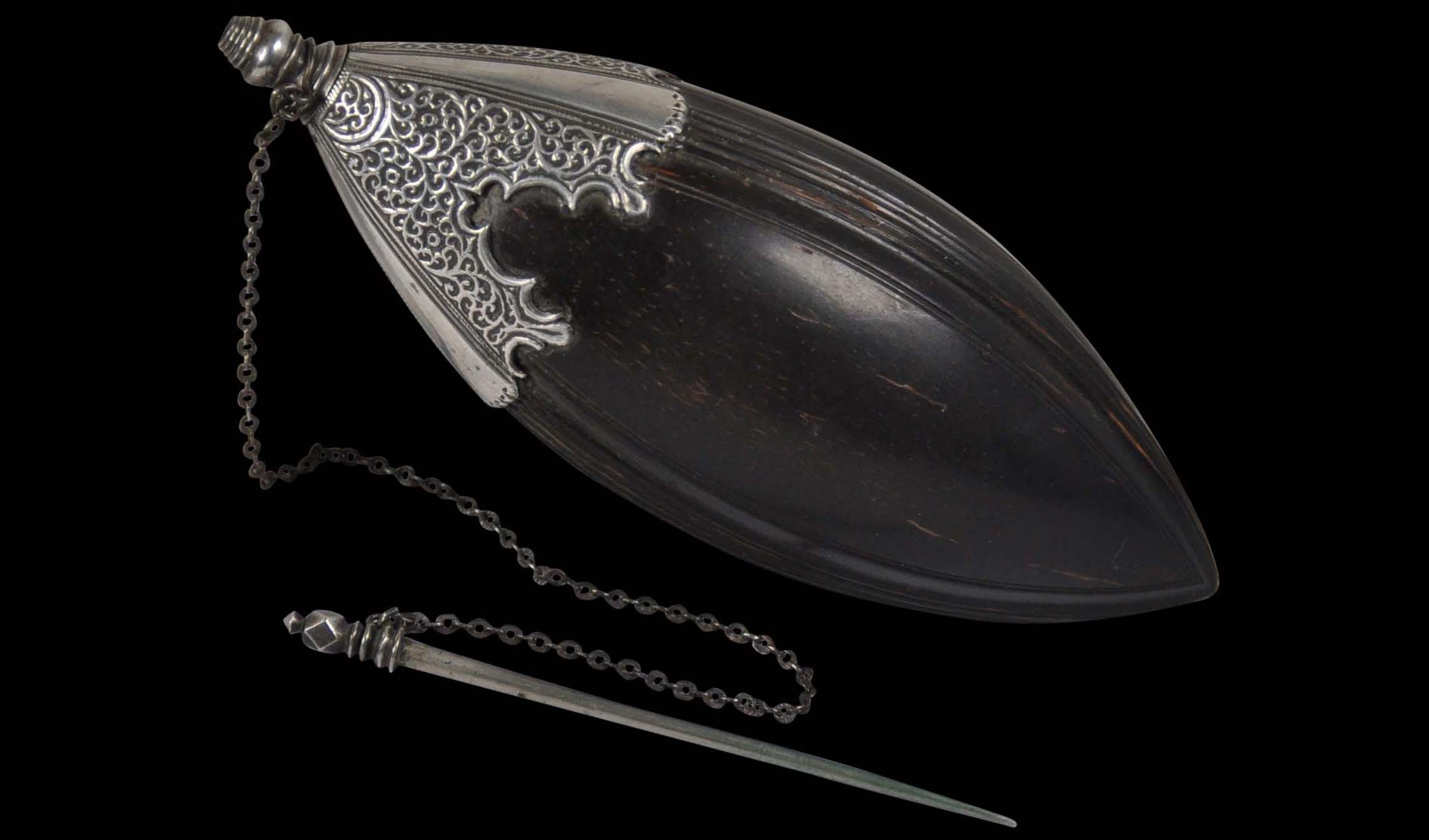This photograph showcases an antique, acorn-shaped container that closely resembles an American football but is more slender. The container appears to be made from wood, evident by the visible wood grain lines beneath the peeling black paint. At the top, there is an intricately designed silver cap, which is connected by a small silver chain to a removable pin or stopper, likely made from metal and resembling a needle. The pin seems to function as a closure or applicator, suggesting the container may have been used to hold a liquid, possibly perfume. The detailed craftsmanship and ornate silver hardware on this unique, dark wooden container hint at its historical and potentially valuable nature.